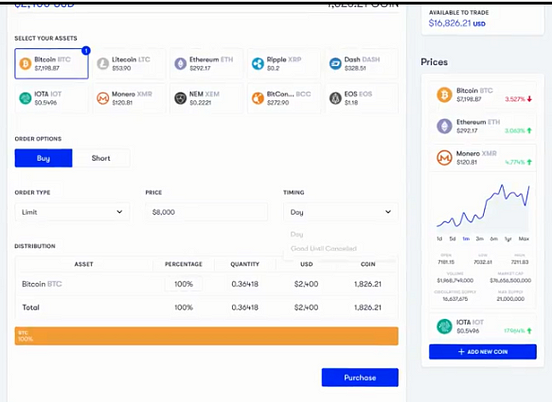The image depicts a computer screen with a trading interface primarily in white. The top of the screen is partially obscured by a black bar, hiding the title of the page. The visible part of the interface features the heading "Select Your Assets," followed by a list of choices, each accompanied by a color-coded circle: one green, several gold, two black, some blue, and one gray.

Below the asset selection section, there are order options, including a blue "Buy" button and a white "Short" button. Users can input their order type via a dropdown menu, specify the price and timing, and then proceed to the "Distribution" section. There's a mention of "Bitcoin Total" under the assets.

A gold bar stretches across the bottom of this section, and beneath it is a blue "Purchase" button. On the right side of the interface is a vertical sidebar with a gray background labeled "Available to Trade." This area displays the number of shares available in US dollars in blue text, with individual stock prices and icons in their respective colors. Below the stock information, a blue graph provides additional details about the stock performance. At the bottom of this sidebar, there's a blue box indicating the option to "Add a New Coin."